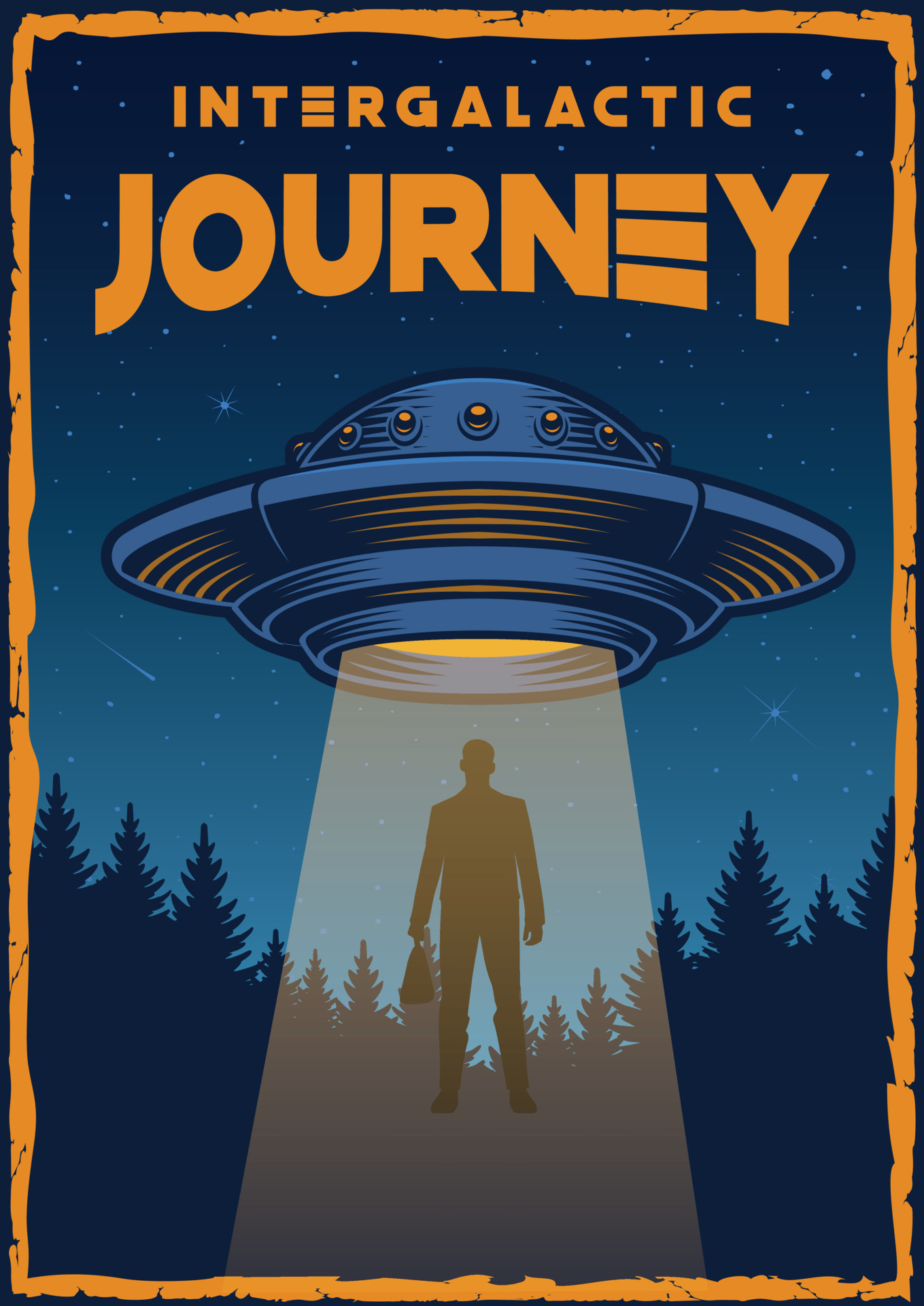This computer-animated poster, with an orange, rugged border and a dark blue and light blue background, depicts a captivating "Intergalactic Journey." The title is boldly displayed in uppercase orange letters at the top, reminiscent of a Star Wars style font, giving it a dynamic, angled presentation. The scene features a night sky studded with bright stars and a shooting star to the left, contributing to the cosmic ambiance. Central to the image is a blue UFO with orange lights, emitting a striking orange beam down onto a silhouetted man wearing a suit and holding a briefcase. The man, seemingly being abducted or lowered, is suspended above shadowy treetops, adding a layer of mystery to his predicament. The entire composition, with its celestial theme and enigmatic elements, resembles a book or magazine cover evocative of a sci-fi adventure, blending elements of suspense and wonder.